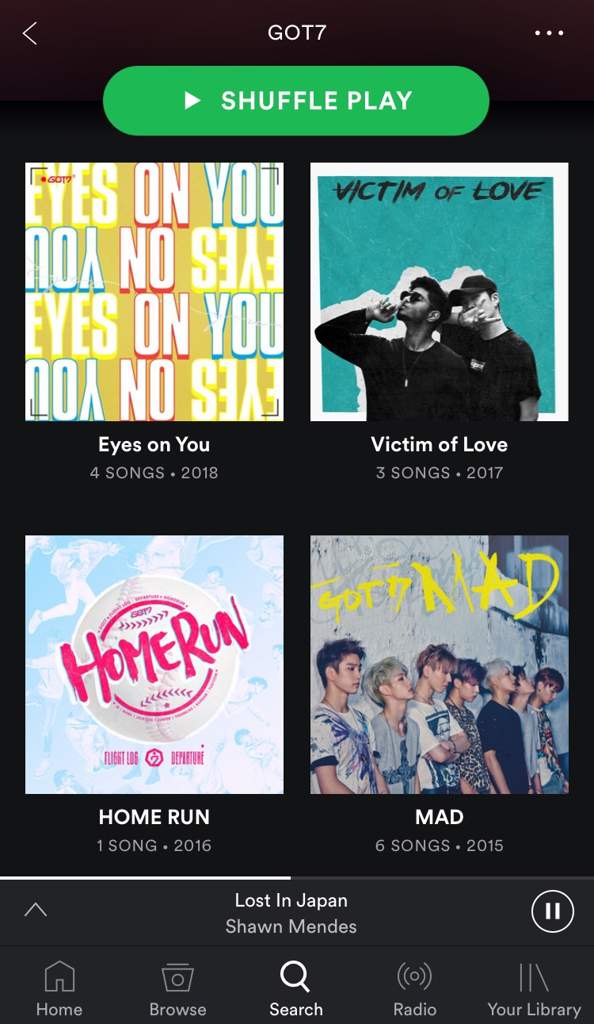Here is a cleaned-up and more detailed version of the caption:

---

This image is a screenshot of a music app on a smartphone. At the top left corner, there is a back arrow pointing to the left. In the top right corner, there are three vertical dots, likely indicating additional options or a menu. Centered at the top, the text "GOT7" is prominently displayed.

Beneath this, there is a green, oval-shaped "Shuffle Play" button with a play triangle icon on the left. Below the button, the screen displays four album covers in a row.

1. **First Album**:
   - **Title**: "Eyes on You"
   - **Background**: Yellow
   - **Text**: The words "Eyes" (white letters with a yellow border), "On" (white letters with a red border), "You" (white letters with a blue border) are written in a peculiar fashion, alternating between being upside down and right-side up.
   - **Details**: "Eyes on You", 4 songs, 2018.

2. **Second Album**:
   - **Title**: "Victim of Love"
   - **Background**: Two young men in black shirts.
   - **Details**: One has his finger to his mouth in a "be quiet" gesture and wears glasses, with black hair. Behind him, another person does a rock-and-roll hand sign, wearing a hat.
   - **Text**: "Victim of Love" (in black)
   - **Details**: "Victim of Love", 3 songs, 2017.

3. **Third Album**:
   - **Title**: "Home Run"
   - **Background**: Faint design of people, with a baseball graphic in the middle.
   - **Text**: "Home Run" (in red letters)
   - **Details**: "Home Run", 1 song, 2016.

4. **Fourth Album**:
   - **Title**: Possibly "GOT MAD" (in yellow letters)
   - **Background**: Seven young Asian men with modern style shirts featuring patterns and splashes of color. One wears a black t-shirt. Hairstyles vary: one has gray hair, one has blondish-brown hair, and the rest have medium to dark brown hair.
   - **Details**: "Mad", 6 songs, 2015.

At the bottom of the screen, the phone's navigation bar is visible. It shows the currently playing song "Lost in Japan" by Shawn Mendes. There are five icons named Home, Browse, Search, Radio, and Your Library.